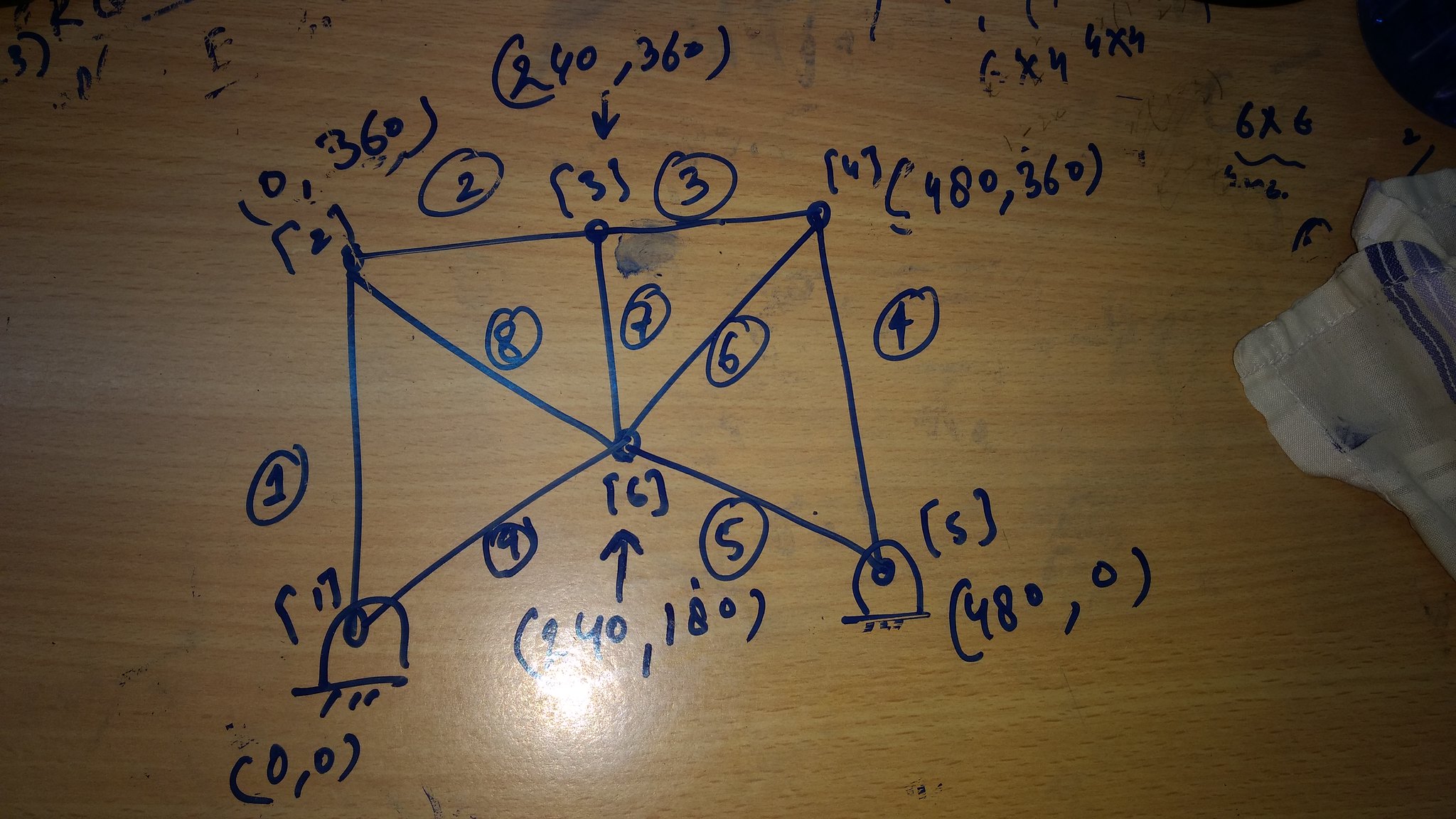The image depicts an intricate drawing created using a blue marker on a brown surface, likely a table or board. The drawing is not done on paper. In the lower right section of the image, there is a white and blue dish rag or washcloth that appears to have some ink stains on it.

The main focus of the drawing is a complex geometric figure consisting of three or four interlocking triangles, with circles at each intersection point. Surrounding this central figure are several numbers encircled with blue marker, including numbers 1, 2, 3, 4, and 5. Inside the triangles, additional numbers such as 6, 7, 8, and 9 are also enclosed in circles.

There are scattered scribbles in the top left-hand corner of the drawing, along with various other scribbles within the same vicinity. Additionally, random numbers enclosed in parentheses are dispersed throughout the drawing.

In the bottom right corner of one of the triangles, the number 5 appears within parentheses. Beneath it, the notation "48 degrees, 0" is written in parentheses. In the bottom left corner of the image, the coordinates "(0, 0)" are marked in parentheses, along with other similar numerical notations scattered around the drawing.